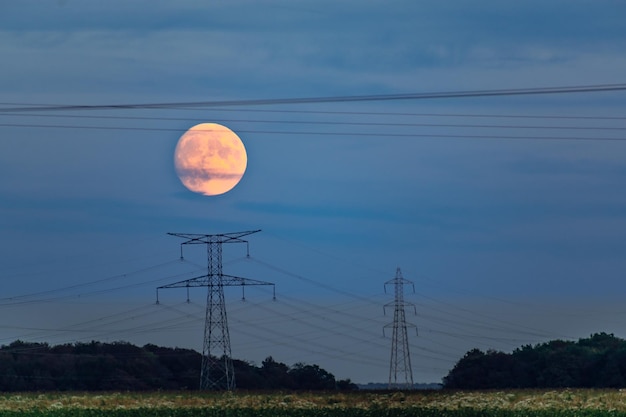In this outdoor photograph set in a rural area, a full, peach-colored moon hangs low over the horizon against a twilight sky that remains light blue. The moon is the largest and most prominent feature, with its craters clearly visible. Beneath the moon, there are two large, black metal cell towers connected by a web of electrical wires, which stretch across the sky and intersect with the moon itself. The scene is framed by grassy fields and scattered trees in varying shades of green, giving a sense of open space. The composition captures the delicate balance of a setting sun and a rising moon, highlighting the intricate pattern of power lines crisscrossing the serene landscape.